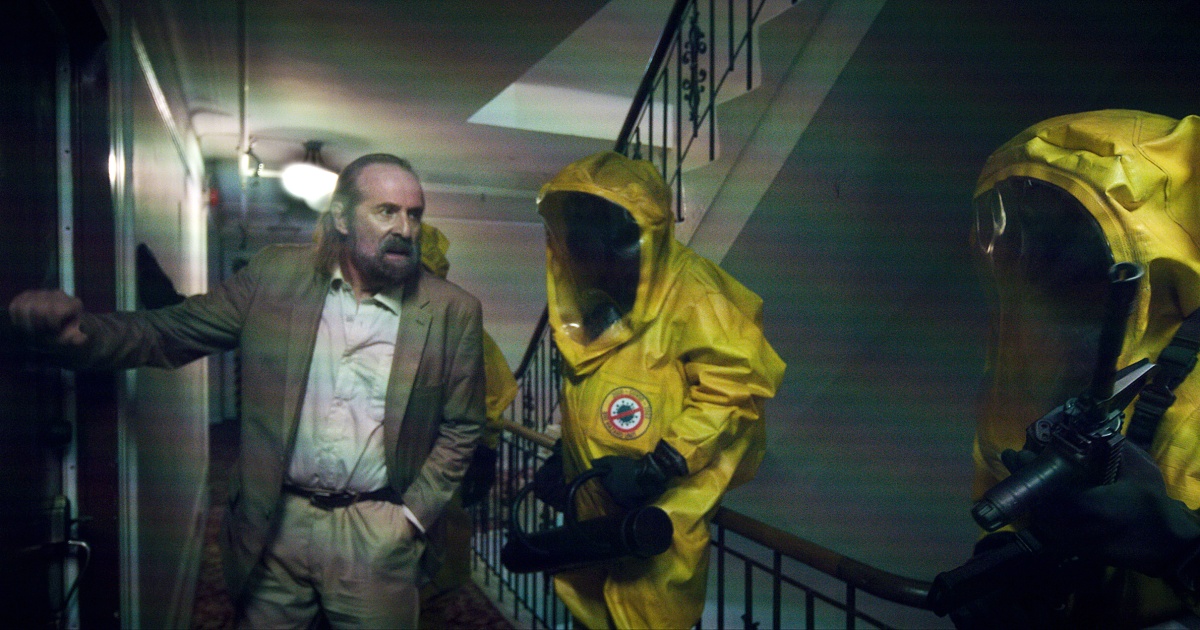In this photograph, an older, desperate-looking man with longish hair and a beard is seen on the left. He wears a brown coat over a white shirt and tan pants, with his right hand extended towards a door as if attempting to knock or open it. He appears to be in a state of distress, speaking to two men on his right who are dressed in full yellow hazmat suits with clear visors and black gloves. The hazmat-suited men are holding what seem to be black instruments, possibly weapons, and are looking intently at the man. The setting suggests an interior location, possibly an apartment or hotel, as indicated by the visible doorways and a metal-railed stairway in the background. The color palette of the scene is mostly composed of grays and tans, contrasted sharply by the bright yellow of the hazmat suits. An emblem on the hazmat suits remains illegible, adding an element of mystery to the scenario which could be a part of a movie scene or a real-life situation.